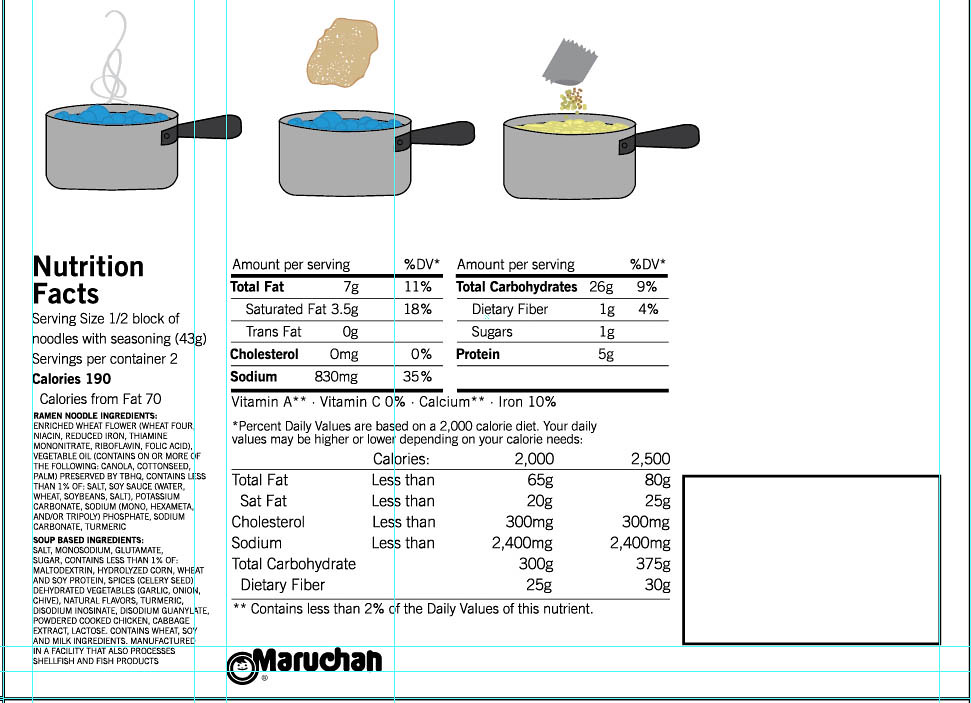The image is a detailed digital rendering of the back of a pack of Maruchan brand ramen noodles, captured in a clean, illustrative style. Prominently displayed at the top are three simplistic, cartoony gray pots with black handles. The first pot on the left shows blue water boiling. The second pot depicts the boiling water with an unwrapped block of noodles hovering above it. In the third pot, the noodles are immersed in the boiling water, with an opened seasoning packet shown sprinkling seasoning into the pot.

Below these illustrated instructions, in clear black print, are sections for nutritional information and cooking instructions. To the lower left, nutritional facts are prominently detailed, with two main categories: total fat and total carbohydrates, each with subcategories of information including calories (190 per serving) and calories from fat (70). Serving size is specified as half a block of noodles with seasoning.

Additionally, extensive ingredient lists for both the noodles and the soup base are located towards the lower left section, embedded into paragraph formats. The name Maruchan, identifiable as the brand, is clearly printed towards the middle left-ish area. The entire design aims to provide a comprehensive overview, ensuring users understand both the preparation steps and the nutritional content.